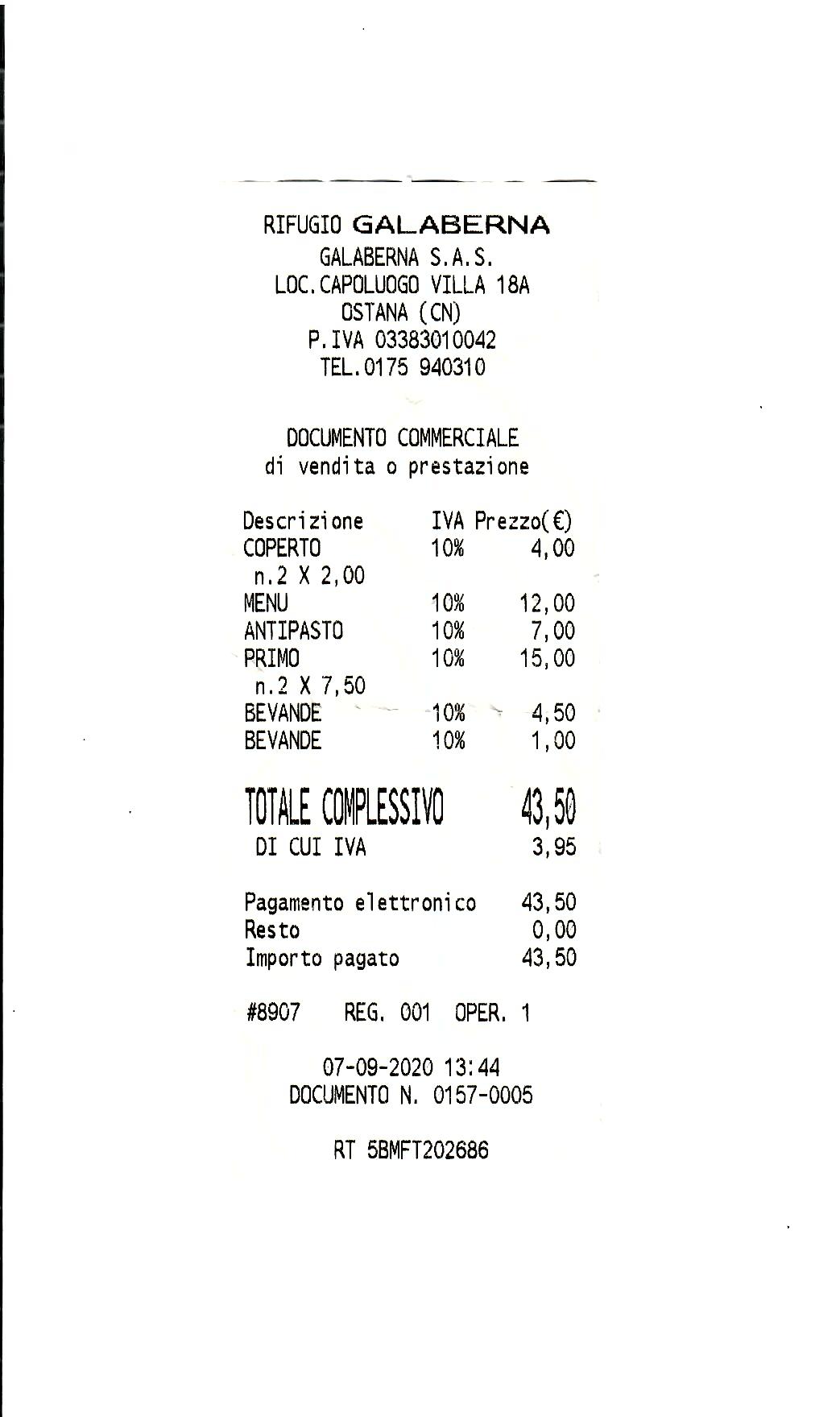This image is a vertically aligned scan of a receipt, predominantly in Italian, with a notable black line running straight down the left side and a minor line at the top. The receipt's header reads "Refugio GALBERNA SAS LOC.CAPO LOGO VIA 18A OSTANA, PIA VIA," followed by contact information. The document is titled "Documento Comerciale di Vendita o Prestazion." The items listed include various categories such as "antipasto" (appetizer), "primo" (entree), and "bavande" (beverages). Prices are displayed to the right, with taxes (IVA) indicated at 10%. The total amount comes to 43,50 euros. The date on the receipt is July 2020. At the bottom, there are several codes including "duplicato," "register," and "documento." The receipt features contrasting black text on a white background, giving it the appearance of a photocopy.